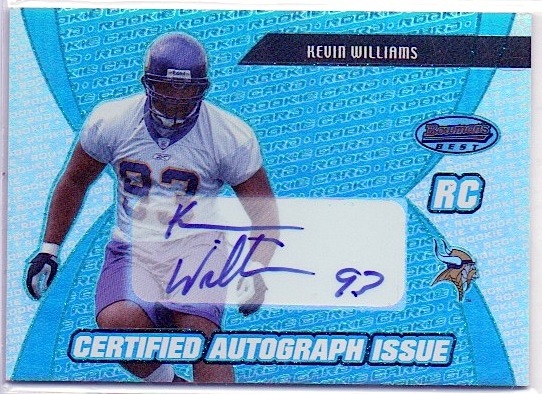This image depicts an autographed football card featuring NFL player Kevin Williams. The card shows Williams mid-run, wearing a white short-sleeved jersey with the number 93, along with matching blue helmet and shorts. His gear also includes gloves. On the right side of the card, the name "Kevin Williams" is prominently displayed, along with the Minnesota Vikings logo, the text "RC," and the logo "Bowman's Best." In the center of the card is Kevin Williams's signature in purple ink, complemented by his jersey number "93." Below the signature, the words "Certified Autograph Issue" are printed. The background features a blue and light blue pattern with the repeated words "Rookie Card."